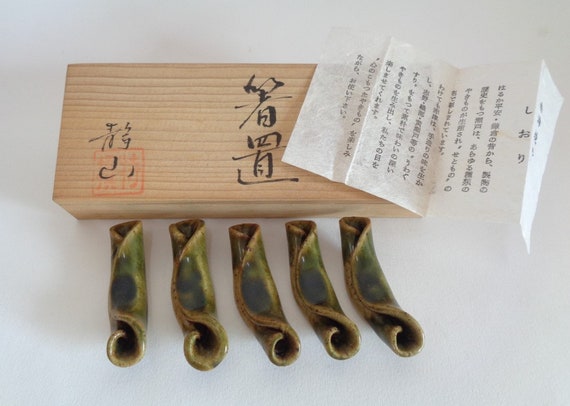The photograph depicts a light-colored, rectangular wooden block, possibly measuring four to five inches long, placed against a white background, which might be a table. A prominent red stamp is located on the bottom left corner of the wood, partially covered by black characters that suggest an Asian language, likely Japanese or Chinese. Additional black characters, larger in size, appear to the right of the stamp.

On the right edge of this wooden block, a thin, translucent piece of white paper, resembling tissue paper, with more Asian characters, lies folded slightly over the edge and dangles off the side. Below the wooden block, five small ceramic objects, reminiscent of folded pieces of dough or rolled-up leaves, are arranged in a row. These objects are tubular and exhibit an earthy color palette, predominantly shades of green, with a darker center and lighter edges. The combination of the wooden block, stamped and written text, paper, and ceramics creates an intricate and visually engaging still life.